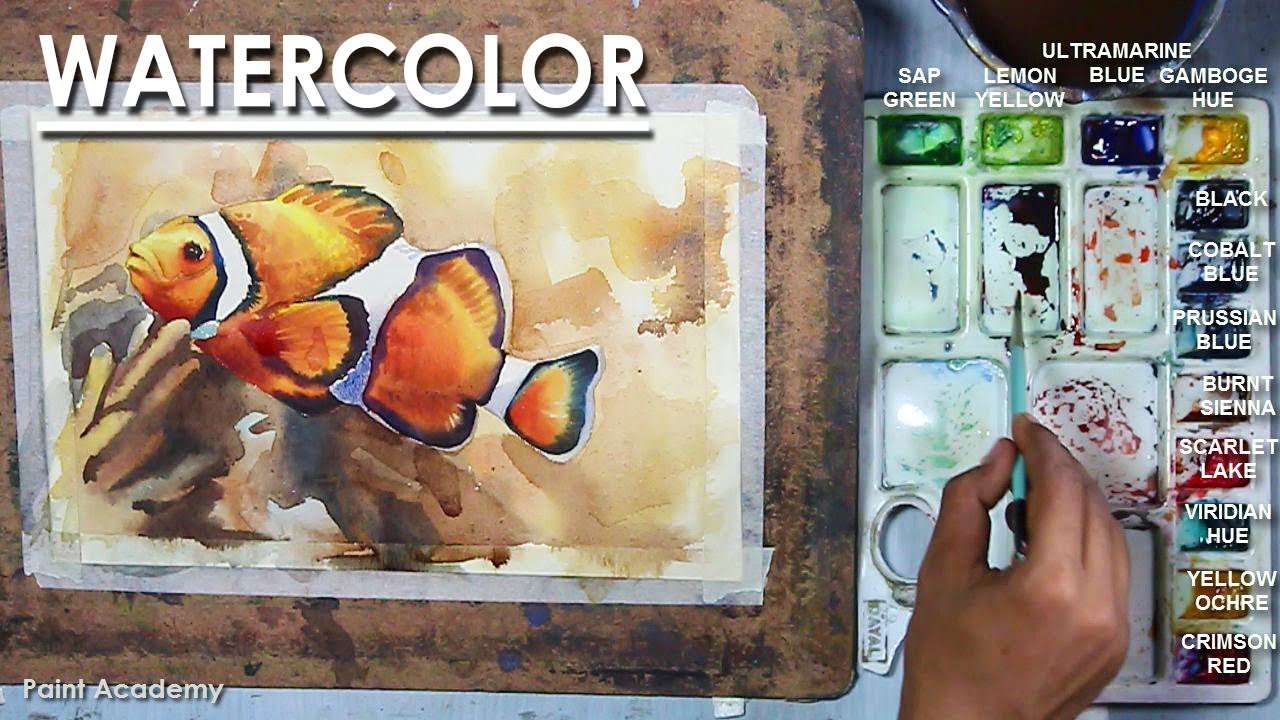The image features a watercolor paint package labeled "Watercolor Paint Academy," with the text "Watercolor" situated at the top left corner and "Paint Academy" at the bottom left corner. The focal point is a vibrant watercolor drawing of an orange clownfish adorned with distinct black and white stripes. Surrounding the drawing are a variety of paint colors displayed on a tray, including sap green, lemon yellow, ultramarine blue, gamboge hue, black, cobalt blue, Prussian blue, burnt sienna, scarlet lake, viridian hue, yellow ochre, and crimson red. Additionally, a light turquoise blue paintbrush is visible, being used to paint. The context suggests that the image may be part of a tutorial or instructional video on watercolor painting.